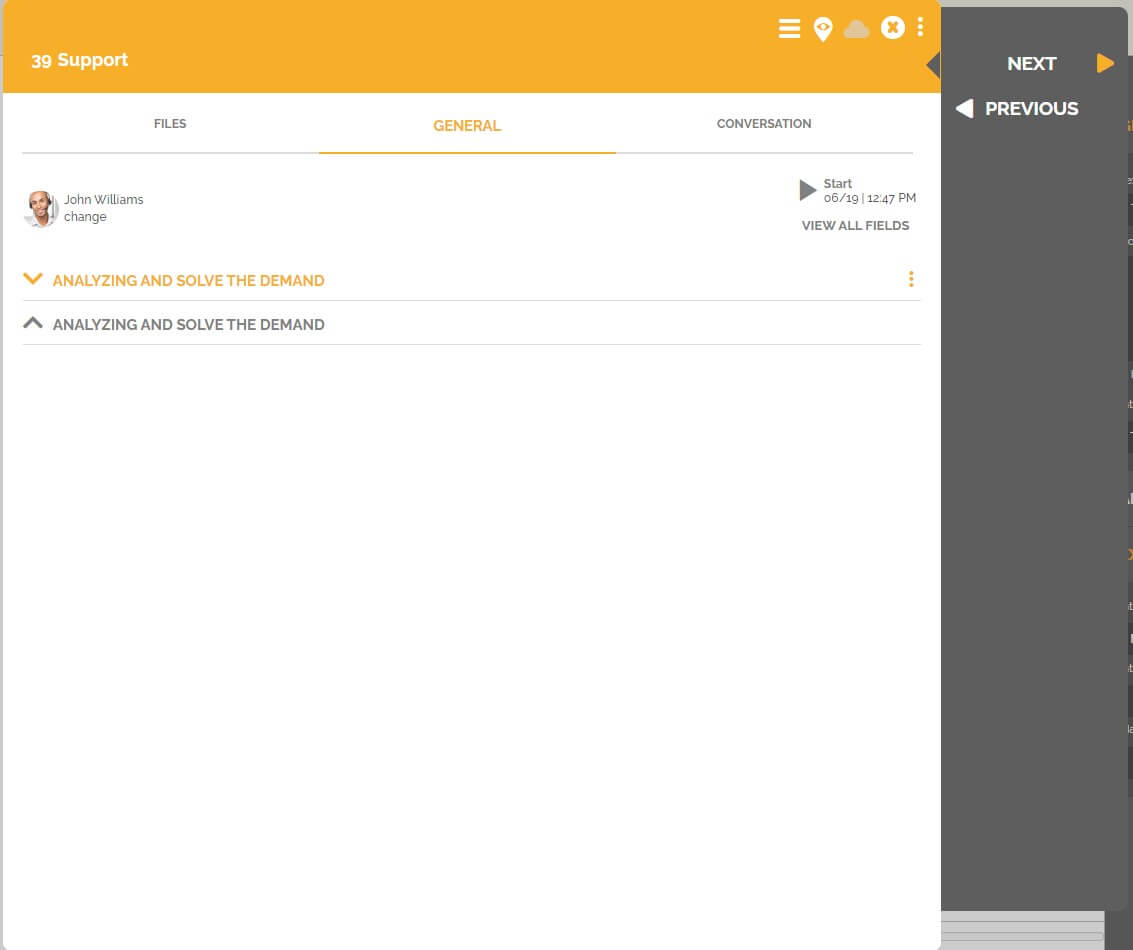The screenshot showcases a webpage for the website "39Support." The top section features an orange title bar with "39Support" prominently displayed on the left in bold text with a capital 'S.' On the right side of the title bar, there are several icons in sequence: a menu icon, a location icon, a cloud icon, a cancel icon, and a more options icon represented by three vertical dots. At the far right, there is a column containing navigation buttons labeled "Next" with an orange right-pointing arrow and "Previous" with a left-pointing triangle.

Directly below the title bar, there are three menu buttons: "Files," "General," and "Conversation." The "General" menu is currently selected, indicated by its highlight in orange and an orange underline. Beneath these menu buttons lies a thin horizontal bar in light gray, spanning the width of the screen.

In the main content area under the "General" menu, the name "John Williams" is shown on the left side. Below this, there is the word "Change." Adjacent to "John Williams" is a profile picture (not described in detail), and to the far right, a gray right-pointing triangle is displayed with the text "Start 06/19 12:47 PM View All Photos."

Further down the screen, the text "Analyzing and solve the demand" appears twice in succession. The overall layout is clean and organized, with key sections and options clearly marked and easily accessible.